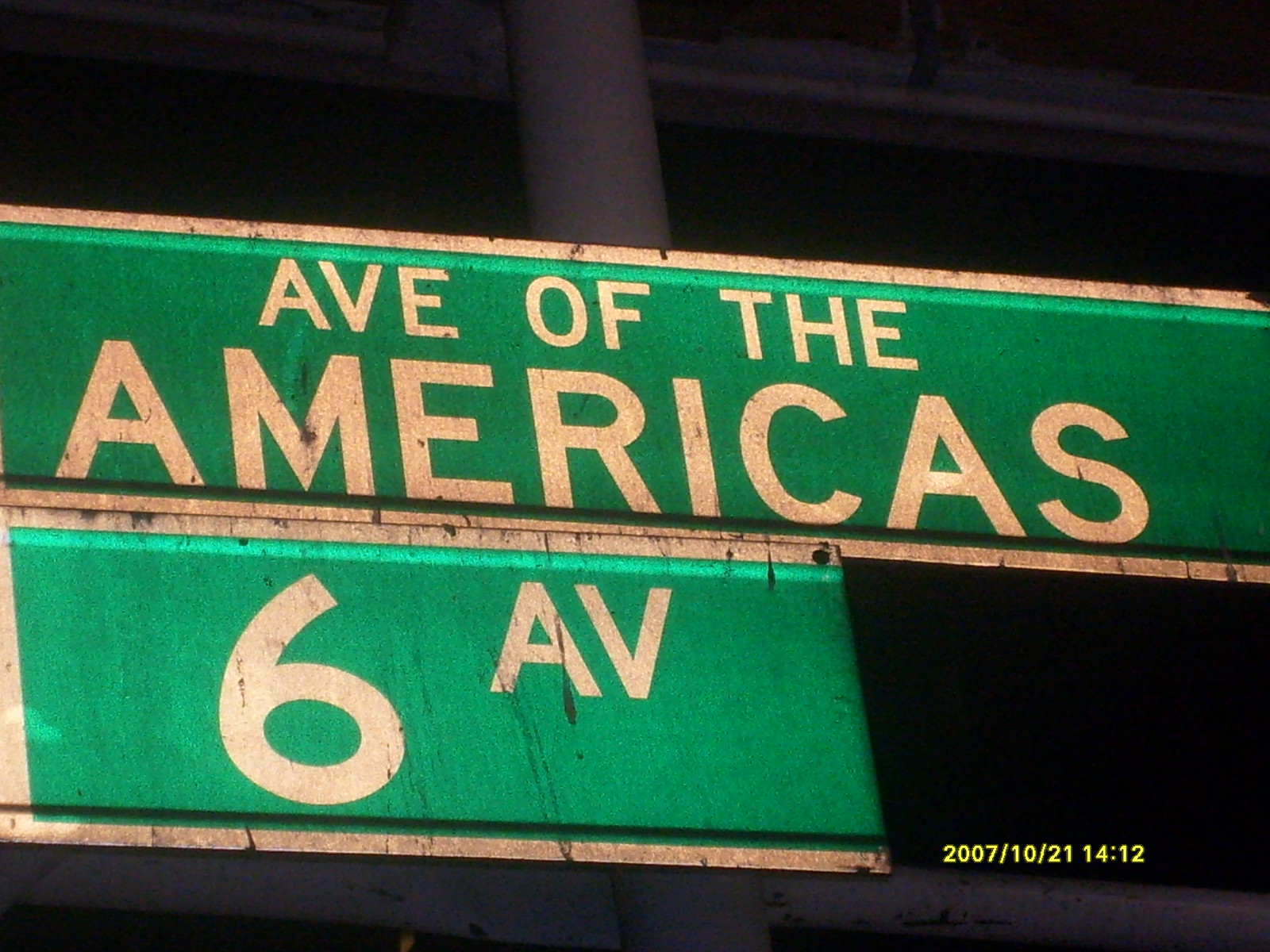This photograph captures a pair of street signs prominently displaying their respective street names. The top sign reads "AVE OF THE AMERICAS" in bold white capital letters, set against a green background with a white border encapsulating the text. Directly below, another sign reads "6 AV," also featuring a green background bordered in white. Notably, the "6" is situated at the bottom of the sign while "AV," in capital letters, is positioned towards the top. The backdrop of the photo is dark, providing a striking contrast to the vivid street signs. In the bottom right corner of the image, a yellow timestamp reads "2007/10/21 14:12," adding a specific historical context to the scene captured.